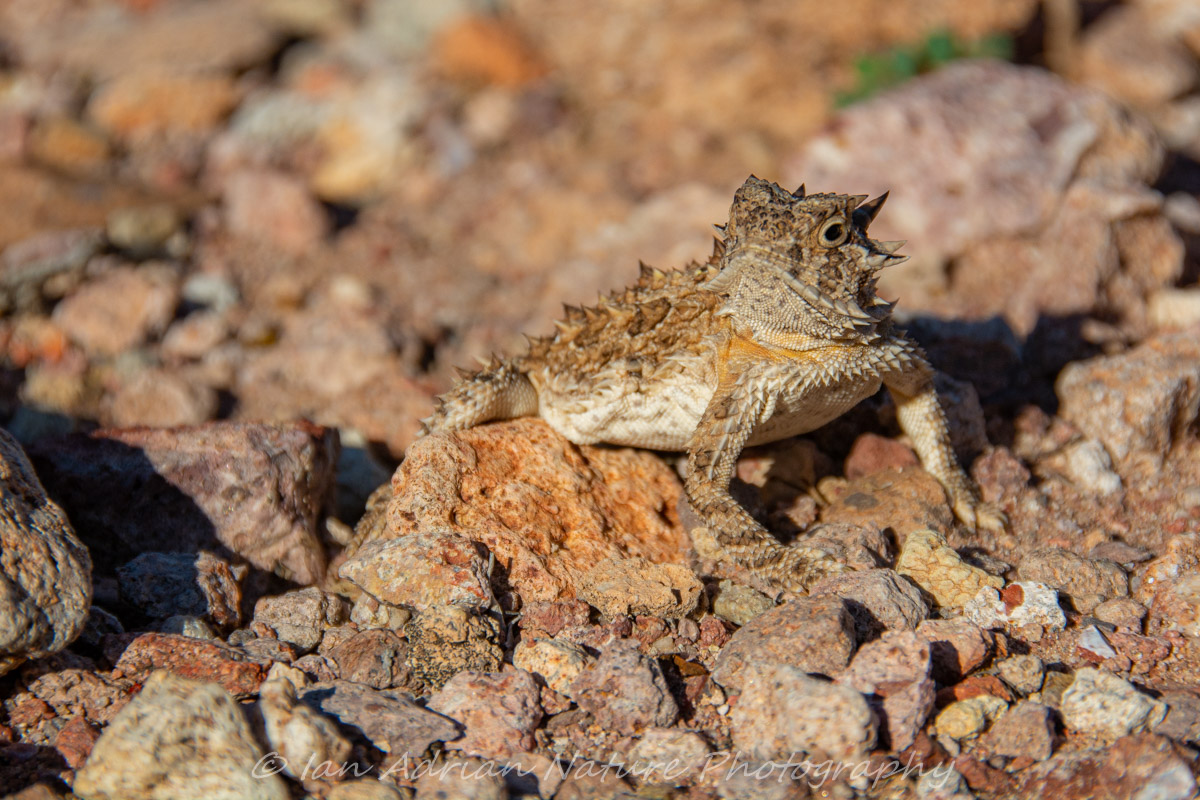This image captures a close-up of a spiky, beige-brown lizard, likely a horny toad, as it stands poised on an assortment of grayish-brown, medium to small rocks in an arid setting. The lizard exhibits a natural camouflage, with its back and face blending seamlessly with the surrounding rocks, which range in color from light brown to dark brown and gray. The creature's lighter, off-white belly contrasts with its upper parts. Its spiky head and body bristle as it looks alertly towards the camera, with its front legs braced and its back belly slightly dragging along the rocks. The photograph features a focused depth of field, emphasizing the lizard while the background blurs slightly. A small patch of greenery is visible behind a larger rock in the upper right corner, adding a touch of color to the scene. The bottom of the image includes white script text reading, "copyright Ian Adrian nature photography," indicating the image was taken during the bright daylight.